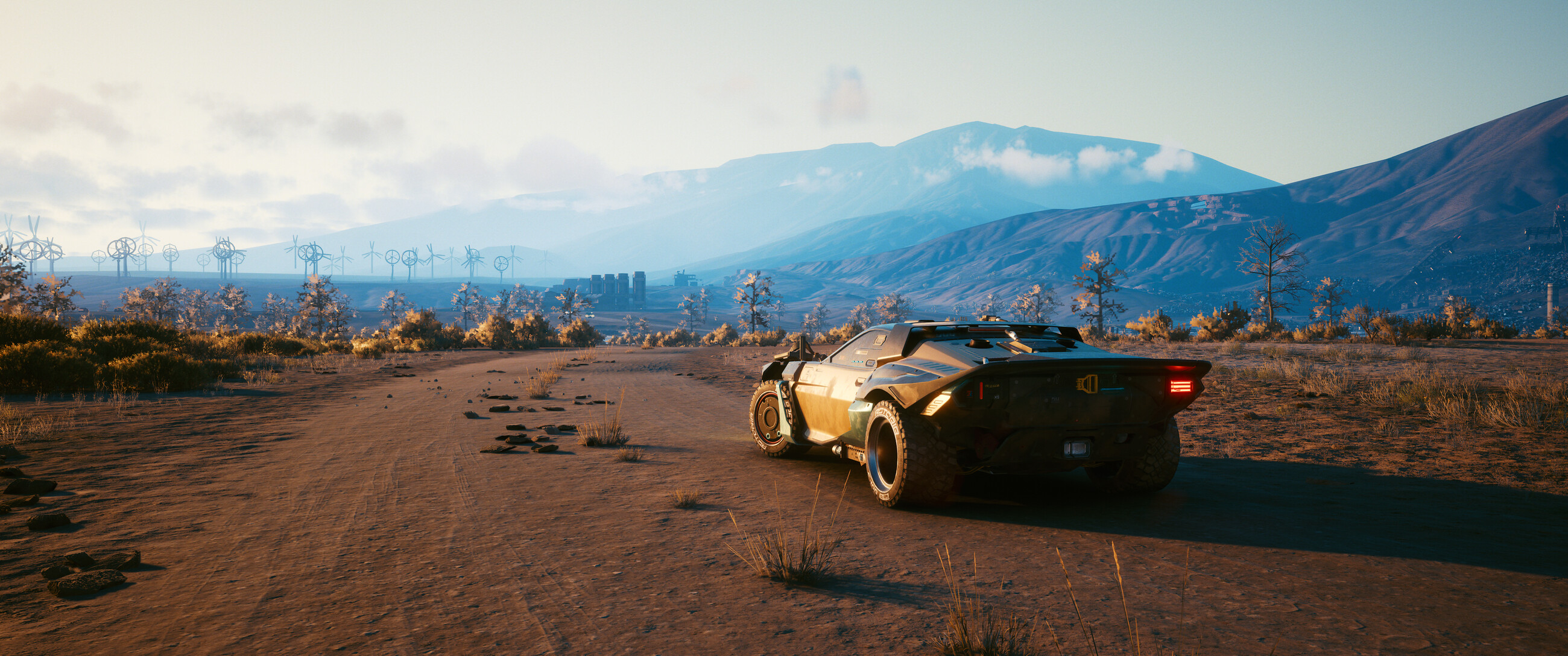This photograph captures a sleek sports car positioned against a rugged desert landscape. The car, a luminous gold in color, stands out with its strikingly large tires and prominent brake lights. The terrain is characterized by patches of sand interspersed with sparse desert vegetation. In the distance, an array of windmills punctuates the horizon, typical of arid environments. The sky above is a clear blue, adorned with scattered white clouds. Although minimal, the presence of desert trees and tufts of grass adds to the authenticity of the scene, illustrating the resilient flora that thrives in such arid conditions.